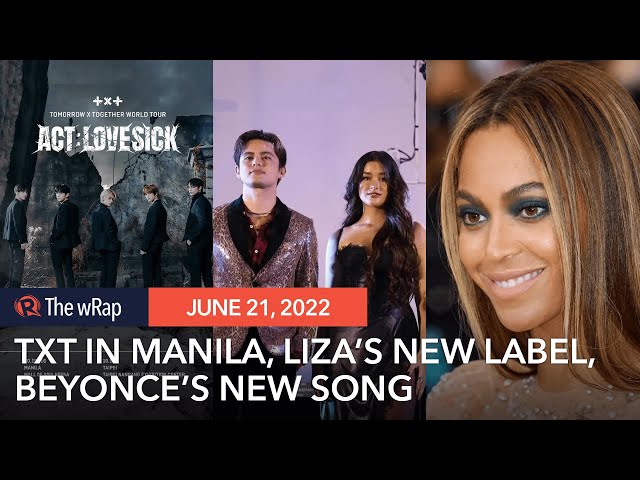A widescreen screenshot of a website called "The WRAP" is displayed, featuring the prominent logo with a red background and a black 'R' angled towards the top left corner. The layout includes three images: the first one, titled "ACT: LOVESICK," features a background picture; the second shows an elegantly dressed couple; and the third is a close-up of a glamorous woman. Adjacent to "The WRAP" logo, there is a rectangular box with white lettering indicating the date "June 21st, 2022." Below the date, the text reads "in Manila, Liza's new label, Beyonce's new song." The website appears to be focused on entertainment news updates and stories.